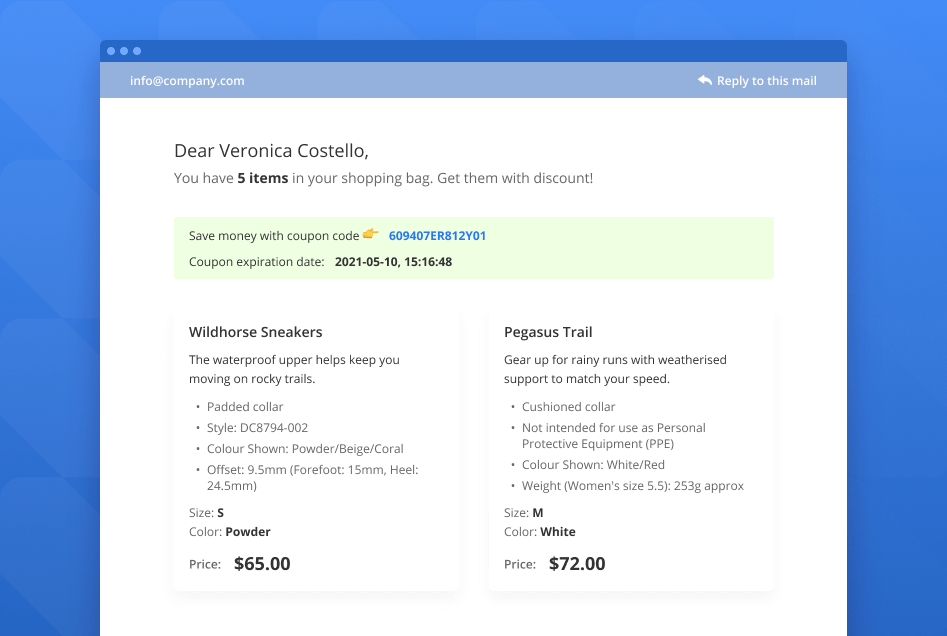The image is a horizontally oriented rectangle featuring a pop-up window or screen at the center. The background is predominantly blue, encompassing the left edge, top, and bottom of the image. Across the top of the pop-up window, there is a dark blue banner with three light blue dots positioned on the upper left.

Directly below the dark blue banner, a light blue banner stretches across the width of the pop-up, displaying "info@company.com" in white text on the far left. Adjacent to this, still within the banner, are a reply symbol and the text "Reply to this email," both in white.

The main section of the pop-up has a white background with predominantly black text. It begins with "Dear Veronica Costello, you have five items in your shopping bag. Get them with discount." The phrase "five items" is emphasized in bold. Beneath this message, a lime green box with black text reads "Save money with coupon code," featuring an illustration of a hand with a finger pointing towards the code, which is displayed in blue. Mentioned below the coupon code is the account expiration date: "2021-05-10, 15:16:48."

At the bottom, the area is divided into two sections. The left section is titled "Wild Horse Sneakers," while the right section is labeled "Pegasus Trail."